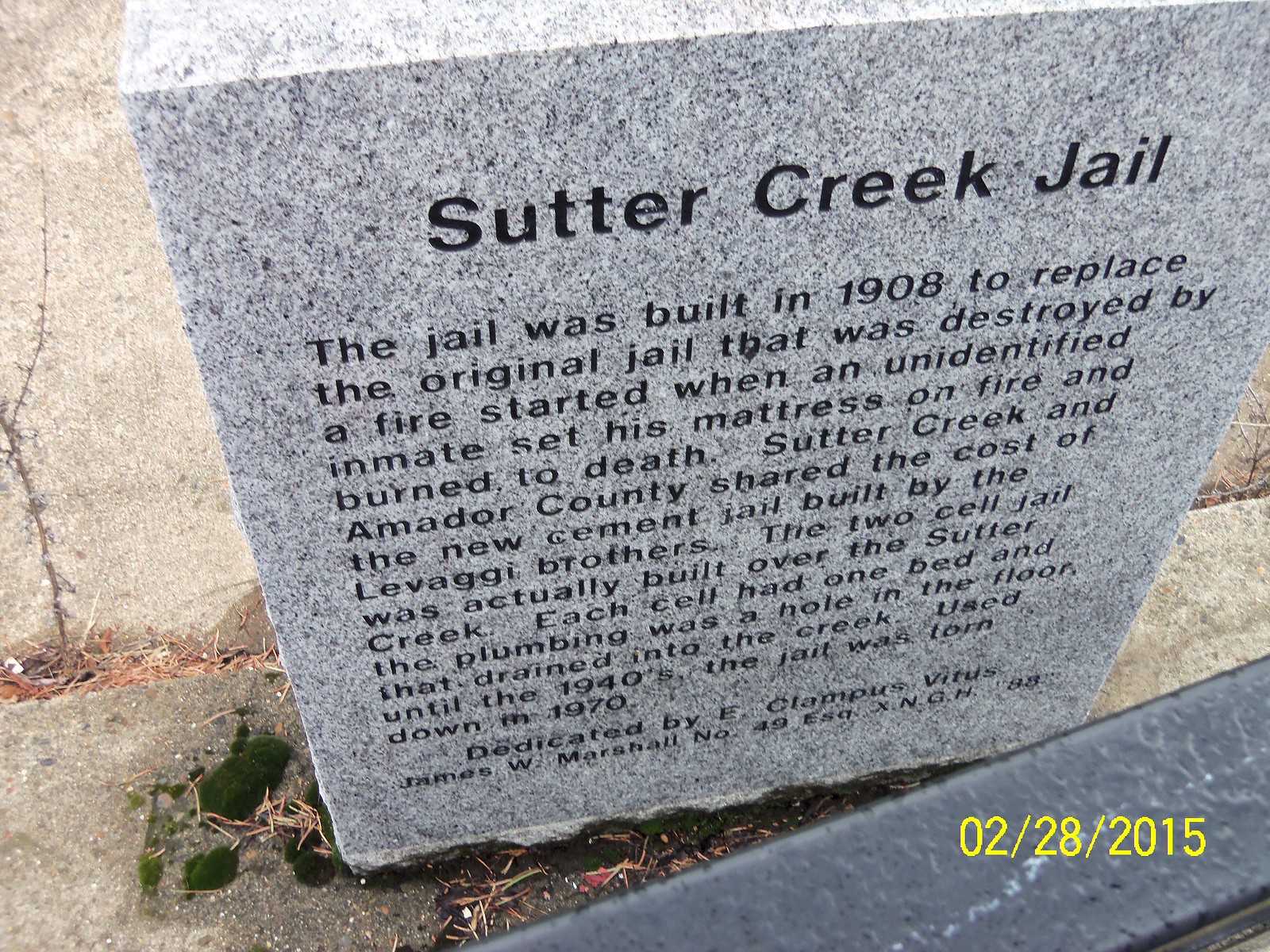The image depicts a historical marker dedicated to the Sutter Creek Jail, crafted from gray stone, resembling a headstone but not for a grave. The stone bears historical information engraved in black text, indicating that the Sutter Creek Jail was constructed in 1908 to replace the original jail, which was destroyed by a fire started by an unidentified inmate who set his mattress ablaze and subsequently burned to death. The cost of the new cement jail was shared by Sutter Creek and Amador County, and it was built by the Levaggi brothers. This two-cell jail was uniquely constructed over the creek, with each cell containing a single bed and primitive plumbing where waste was disposed of through a hole in the floor draining directly into the creek. The jail remained in use until the 1940s and was ultimately demolished in 1970. The bottom right corner of the marker includes a dedication by the historical organization E Clampus Vitus, James W. Marshall Chapter No. 49, and displays the date "02-28-2015" in yellow, indicating when the photo was likely taken. The scene is set against a light gray sidewalk with visible cracks and some moss in the bottom left corner, adding to the weathered historical context.